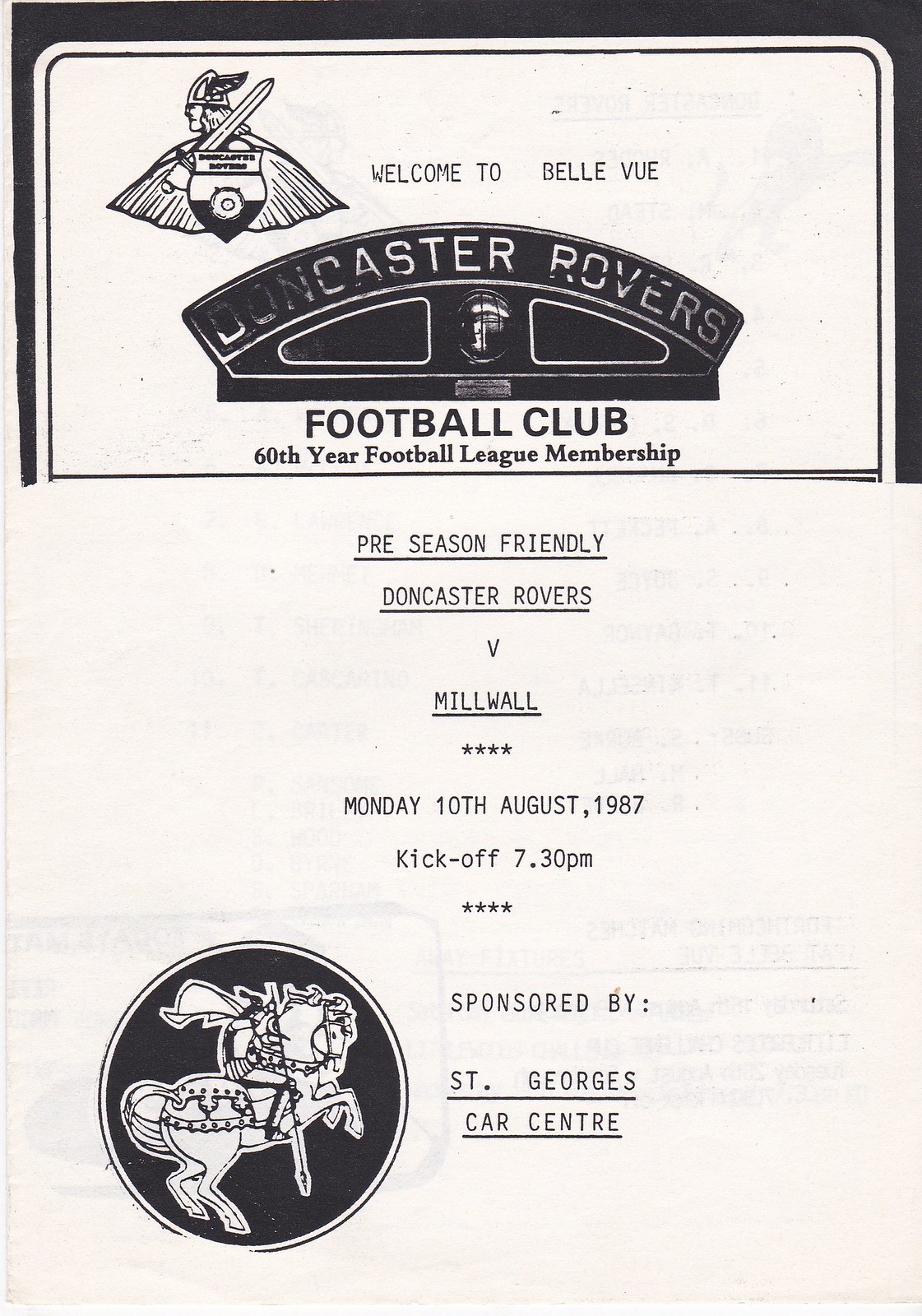The black-and-white cover of this game-day program showcases a mix of historical and event-specific details. At the top, the cover hails, "Welcome to Belleville" next to a small logo on the left, possibly depicting Hermes or Mercury holding a sword, adorned with a winged helmet. The larger central text announces, "Doncaster Rovers Football Club 60-Year Football League Membership." Below that, the main body of the page details a preseason friendly match, reading, "Doncaster Rovers v. Millwall, Monday, 10th August 1987, Kick-off: 7.30 p.m." The event is sponsored by St. George's Car Center, indicated at the bottom center of the poster. In the lower left, a black circular logo features a depiction of St. George on a rearing horse, brandishing a sword. The overall design suggests that the bottom half might be a newer addition, overlaid on an older template to update event-specific details.